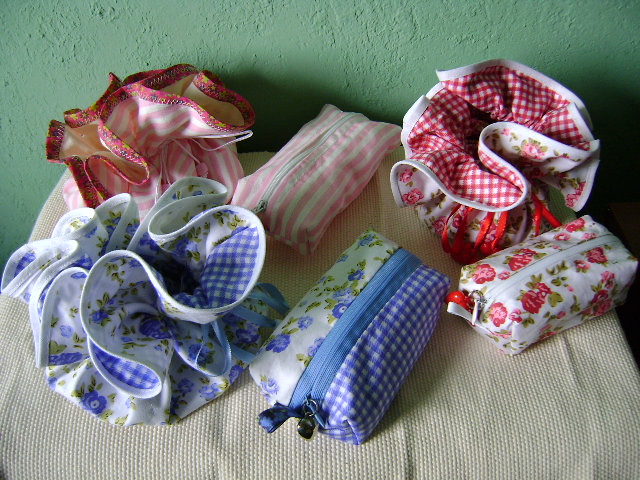This color photo showcases an assortment of hand-sewn toiletry or makeup bags arranged on a nubbly, pale green and white linen tablecloth, set against a light green painted wall background. The foreground features three sets of fabric containers, including rectangular zippered bags and matching cinch bags with pull strings. The first set includes a bag with a white background adorned with little red or pink flowers and a complementary cinch bag featuring the same fabric and red gingham interior, alongside a red satin pull string. The second set displays a blue-themed pattern with one side of the rectangular bag covered in blue gingham, the other side featuring blue forget-me-not type flowers on a cream background, and a matching cinch bag with the same floral exterior and gingham interior, accompanied by a blue zipper. The final set showcases a white and pink striped bag with a pink zipper and a coordinated cinch bag with a white satin pull string. Each zippered bag features a functional design with zippers running lengthwise and small loops for easy handling.